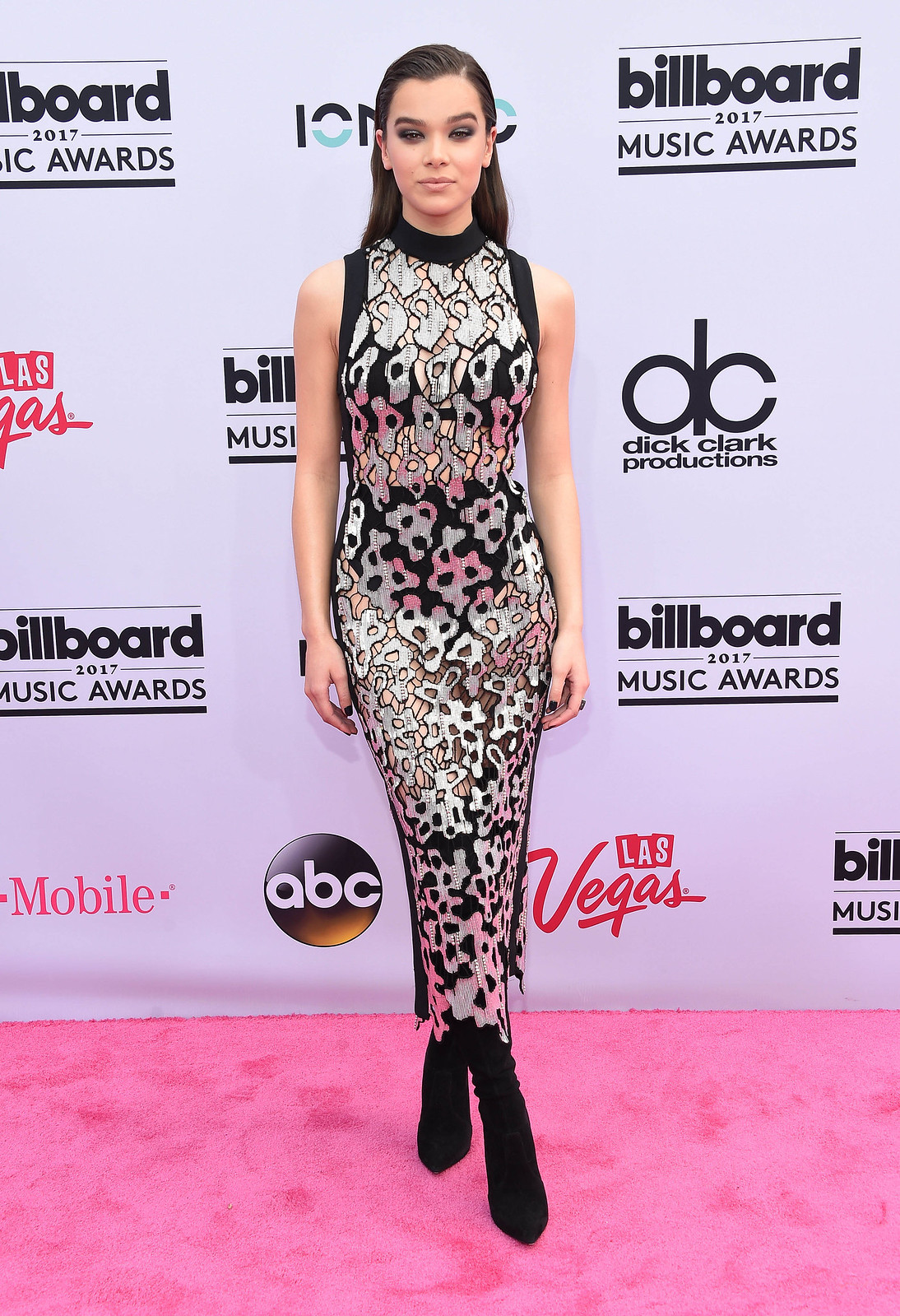In this striking photo from the 2017 Billboard Music Awards, actress and singer Hailee Steinfeld dazzles on a plush pink carpet, positioned in front of a white backdrop featuring the event's logos, including Billboard, ABC, and T-Mobile. Steinfeld, noted for roles in movies and the TV show "Hawkeye," is a young, glamorous white woman with long, brown hair styled back and slightly gelled. She wears a semi-transparent, form-fitting black dress adorned with silver, pink, and light yellow details, highlighting a reflective pattern that accentuates her appearance. Her black high-heeled boots complement the outfit perfectly. Standing alone with one foot subtly crossed in front of the other, Hailee strikes a poised yet approachable stance, her arms relaxed by her sides. Her makeup features smoky eyeshadow, and she offers a half-smile with her eyes slightly squinted, exuding confidence and elegance.